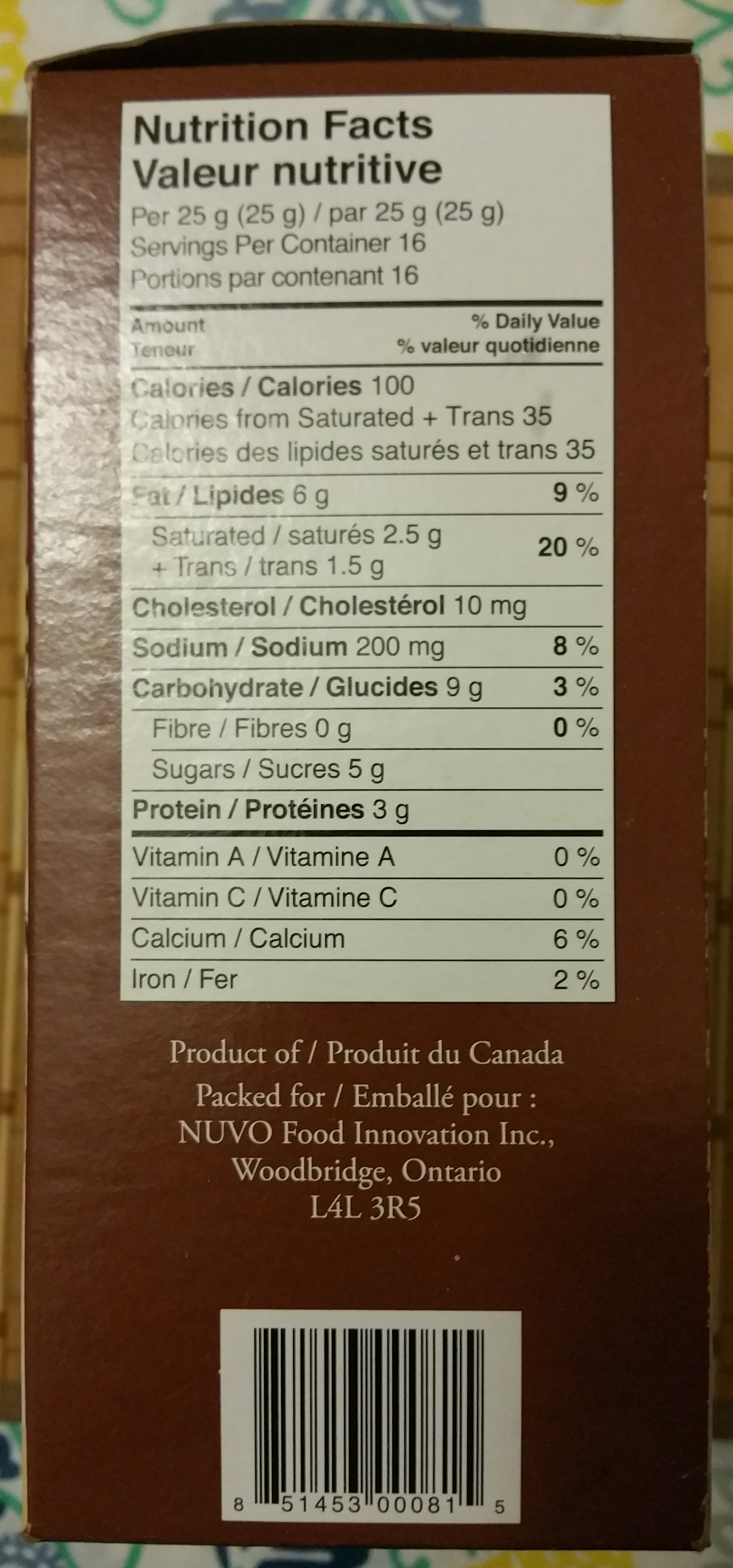The side of a box containing a food item is meticulously detailed in both English and French languages, reflecting its Canadian origins. At the top of the box, prominently displayed, are the words "Nutrition Facts" and "Valeur Nutritive," indicating detailed nutritional information. This bilingual packaging includes details such as the calorie content, which is spelled identically in both languages. 

Located at the bottom of the box is the indication "Product of/Produit du Canada," clarifying the product's Canadian origin. The package originates from Woodbridge, Ontario, produced by Nouveau Food Innovation, a detail highlighted on the packaging despite the actual contents of the box being unknown. 

The box itself is a reddish-brown color with an off-white inset panel occupying the top two-thirds of one side, where all nutritional information, including cholesterol and sodium levels, is meticulously listed. A barcode is visible at the bottom of this panel, with a check digit of eight on the left and five on the right, followed by the numbers 81453000081, which can be used to identify the specific contents of the box.